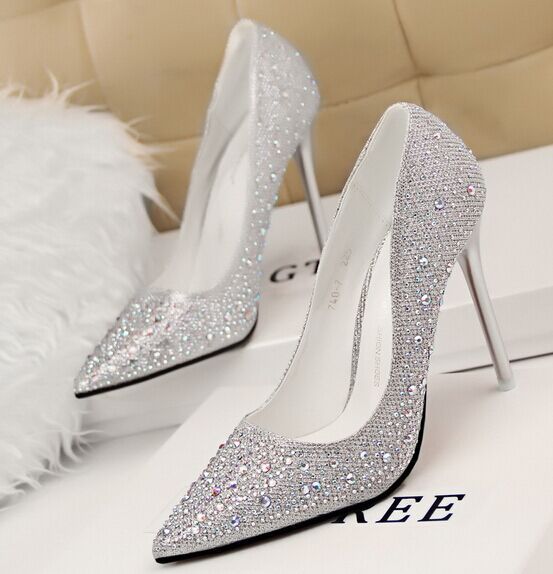This photograph showcases a pair of extravagant, highly embellished stiletto high heels displayed in an elegantly detailed setting. The shoes, featuring sharply pointed toes, are encrusted with various sizes of silver rhinestones that sparkle brilliantly. They boast a sleek metallic or silver post, standing on glossy black soles, and are lined with a pristine white interior. The heels are positioned diagonally, with one shoe slightly elevated on a stack of thin white shoe box lids that bear partially obscured black text, showing visible letters including "GG," "R-E-E," and "GT." Beneath these boxes lies a flat white fabric, while the background features a richly textured, pleated brown leather cushion with a quilted pattern. Adjacent to the shoes is a soft, white feathery object, possibly a pillow, adding a touch of whimsy to the sophisticated display.